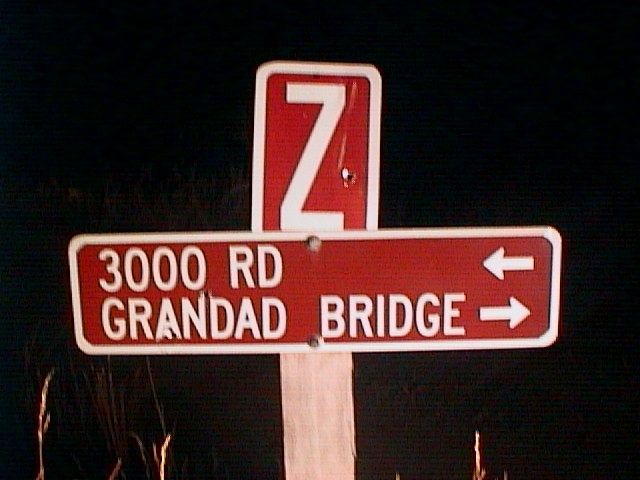This nighttime outdoor photograph captures a street sign mounted on a weathered wooden post. The signpost supports two signs arranged in a plus-sign formation. The upper, vertically aligned sign is a red rectangle with a white border and features a prominent white capital letter "Z." The sign appears damaged, possibly punctured, near the lower right of the "Z." Below this, a horizontally aligned sign also bordered in white reads "3000 RD" in capital letters on a white background, with an arrow pointing to the left. Directly beneath, another segment of the sign reads "GRANDAD BRIDGE," also in capital letters, with an arrow pointing to the right. The lower portion of the sign is bolted to the post, and this section shows signs of wear, including potential bullet holes or punctures over the word "Grandad." Illuminated by the camera's flash, the foreground includes a few stalks of tall grass, while the background remains entirely black, emphasizing the isolation and stark contrast of the illuminated signposts.